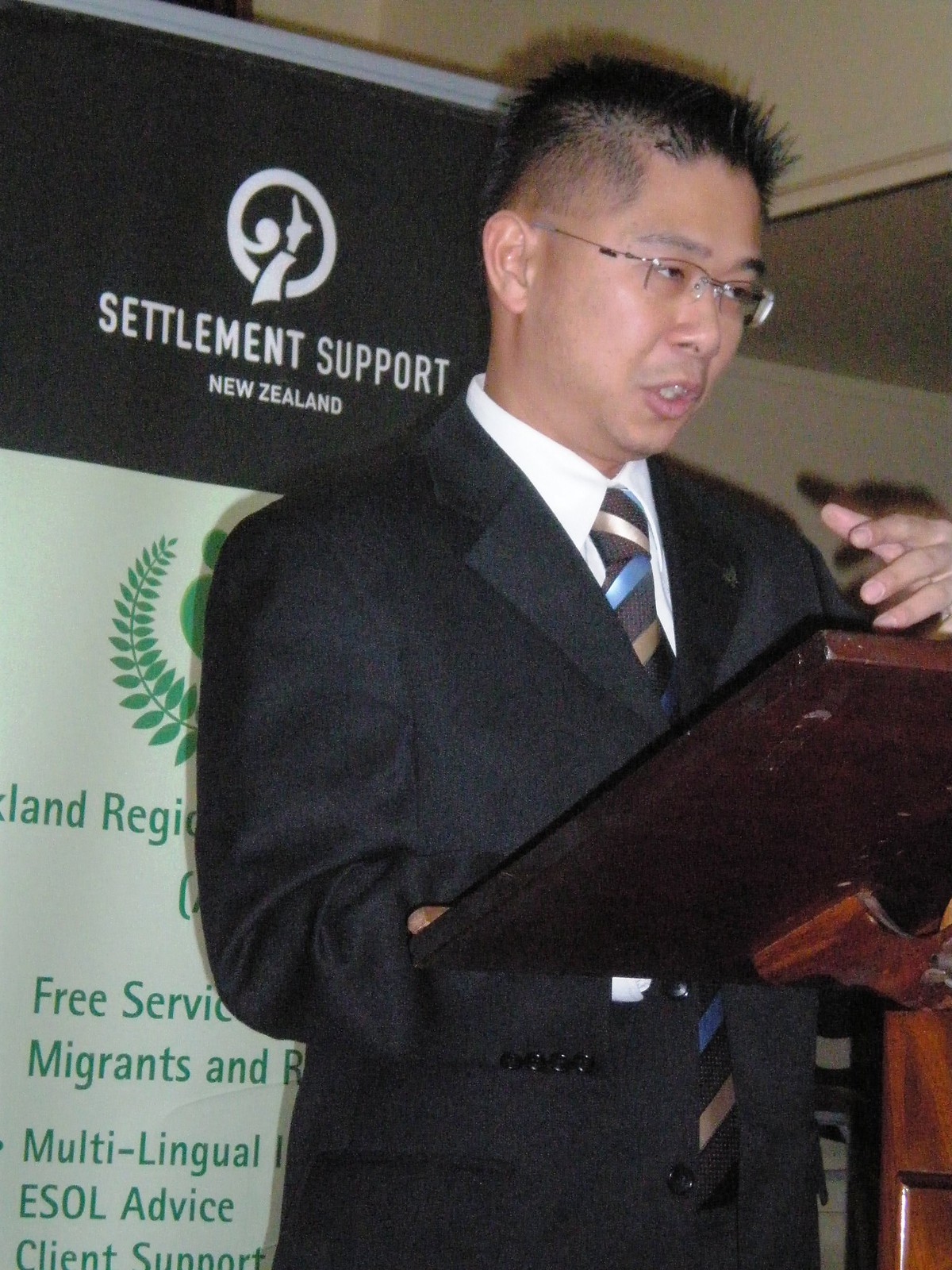The image depicts a young Asian man, likely in his 30s, standing at a dark brown podium and addressing an audience. He is dressed in a black suit with a white shirt, complemented by a tie featuring cream, blue, and brown stripes. The man has short, spiked black hair and is wearing wire-rimmed glasses. He appears engaged in his speech, gesturing with his left hand. Behind him is a black and white banner displaying the text "Settlement Support New Zealand" and some additional details about the services, including terms like "free service," "migrants," "multilingual," "ESOL advice," and "client support," potentially mentioning the Auckland region. The overall scene conveys a formal and professional setting, likely a seminar or conference related to migrant support services in New Zealand.